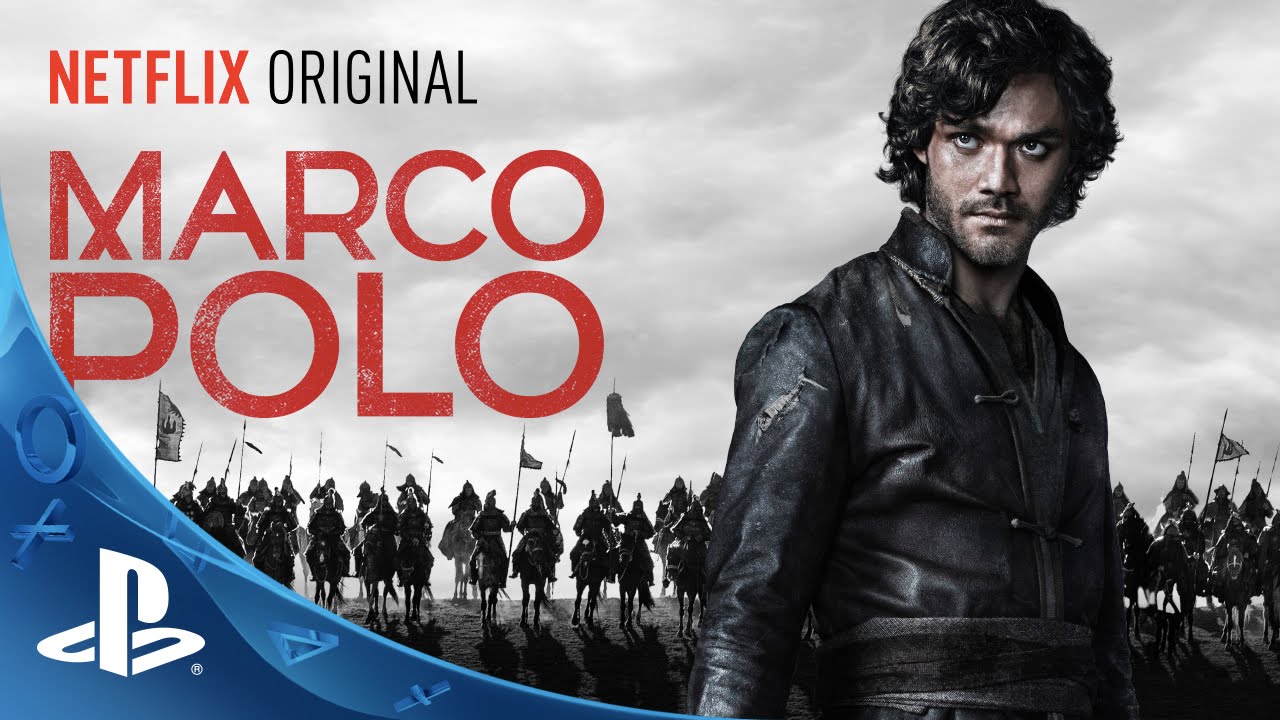The image is an advertisement for the Netflix original series "Marco Polo". Dominating the top left corner are the words "Netflix" in red and "Original" in black, with "Marco Polo" in large red letters beneath them. The central focus of the image is a man with medium-length, bushy black hair, wearing a black leather jacket. His intense gaze is directed towards the upper left. He has tan skin and appears to have a stubbly mustache and beard. Behind him, under a gray, overcast sky, stretches a black ground. A row of cavalrymen, clad in what looks like armor, ride horses across the scene; they carry spears adorned with flags. A blue area in the bottom left corner features the PlayStation logo in white, along with blue Xs, Os, triangles, and a plus sign.